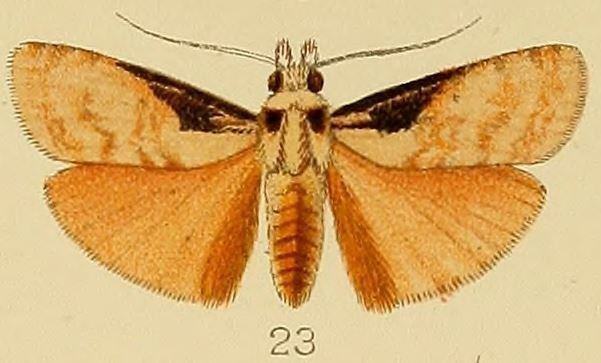The image features a detailed, semi-realistic drawing of a light brown moth with prominent dark brown markings. The moth is viewed from the front, displaying its large, dark brown eyes and two long, curved antennae. The tan or cream-colored background adds a subtle contrast to the insect's light brown body, which has darker brown patches near the eyes and on the upper wings closest to its head. The wings, spread out to their full extent, show intricate folds with fuzzy or fluffy edges, and darker brown areas are also noticeable towards the abdomen and on the tail. The upper part of the moth's body appears to have some fuzzy protrusions. At the bottom of the image, the number "23" is visible, perhaps serving as an identifier, suggesting this could be part of a classification or species diagram. The image has a slightly pixelated, aged look, hinting that it might be an older illustration.